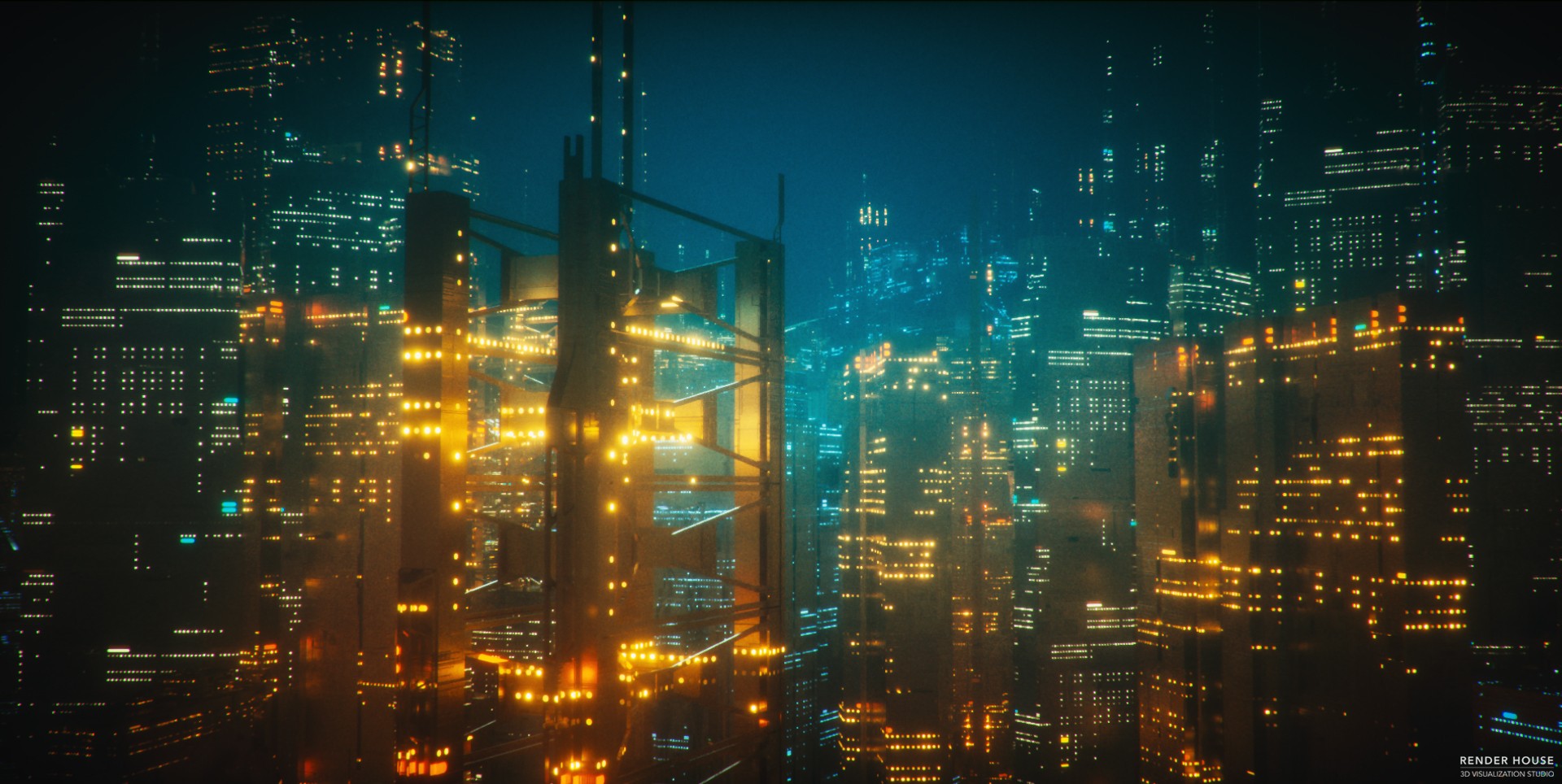The image captures a bustling metropolis at night, dominated by an array of high-rise buildings with rows upon rows of illuminated windows. The nighttime sky provides a deep, almost black, backdrop with dark blue hues. The buildings are tight-knit, forming a dense urban jungle, and their angular, rectangular shapes and straight lines create a sharp, modern aesthetic. Many tops of the skyscrapers are adorned with spindles or pointed structures, adding to the dramatic silhouette against the dark sky. The image is tone-rich, featuring a striking balance of golden and teal lighting, casting a classic contrast of highlights and shadows. In the bottom right-hand corner, the text "Render House" in white all-caps identifies the image's source. The photograph is a horizontal, rectangular frame focusing solely on the buildings and their lights, leaving the street level out of view.